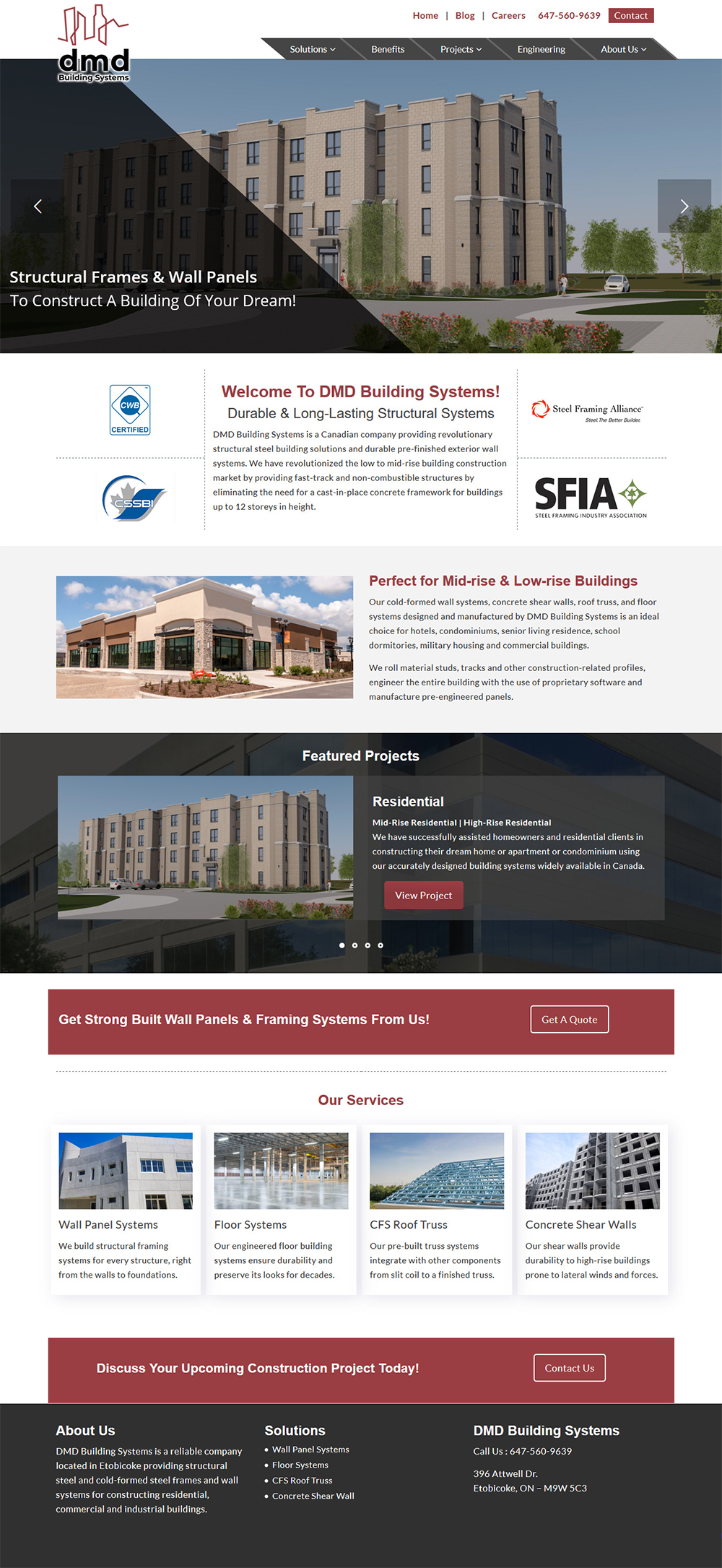![DMD Building Systems Website Overview]

The DMD Building Systems' website features a comprehensive navigation layout designed for easy access to various sections of the site. The website's logo, a continuous line drawing of skyscrapers, sits prominently above the main title "DMD Building Systems." The top navigation bar includes straightforward options: Home, Blog, Careers, a phone number, and a Contact button, all of which direct users to the relevant pages.

Directly below the main navigation, secondary navigation boxes are displayed, including Solutions, Benefits, Projects, Engineering, and About Us. The top frame of the website showcases an image of four-story buildings, likely apartments or office buildings, with the tagline "Structural frames and wall panels to construct a building of your dream" superimposed on a black triangular box.

Beneath this introductory section, the page is divided into seven horizontal information boxes, although the detailed text is quite small and challenging to read. The first of these sections welcomes users to DMD Building Systems, highlighting their durable and long-lasting structural systems. It also shows affiliation logos, with the Steel Framing Alliance (SFIA) being notably visible.

The second section promotes their structural systems as "Perfect for mid-rise and low-rise buildings," accompanied by an image of a one-story, corner-store looking building. Following this, the "Featured Projects" section displays the same four-story building from the top image, categorizing it as a residential project and inviting users to view the project details.

Further down, a section dedicated to quotes encourages visitors to "Get strong build wall panels and framing systems from us." This is followed by the "Our Services" section, which outlines specific services offered: wall panel systems, floor systems, CFS (cold-formed steel) roof trusses, and concrete shear walls. Each service box includes clickable descriptions and images.

Towards the end of the page, another strip prompts users to contact DMD Building Systems to "discuss your coming construction project today." Finally, the page concludes with a black box containing essential information about the company, including sections on About Us, Solutions, contact details, and location information.